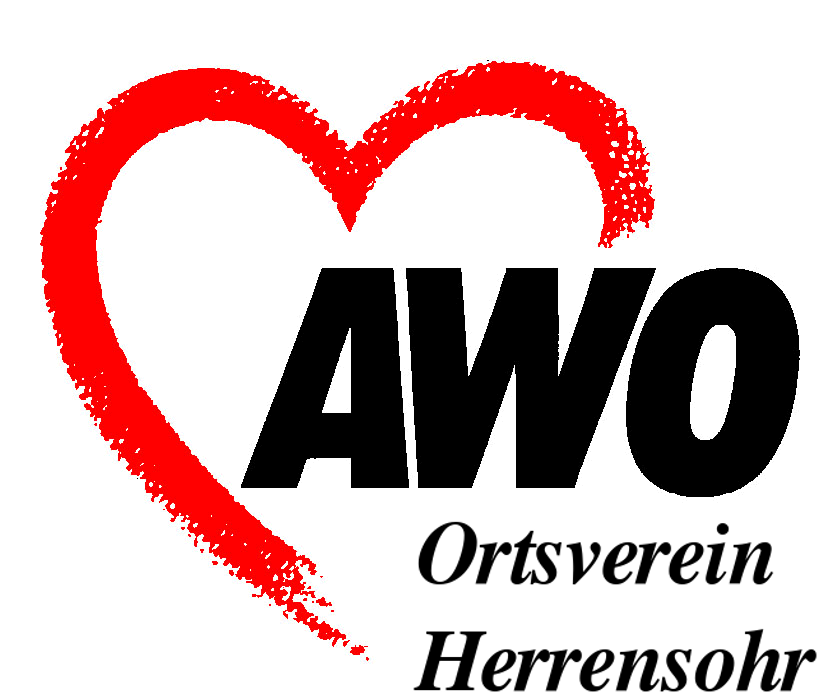The image showcases a logo against a pure white background that creates a floating effect for the elements within. The logo is dominated by a hand-drawn heart positioned in the top left. This heart has a unique painted appearance, with a striking red outline and a white interior. Centrally located are the bold black letters "A-W-O." Directly below this, in a separate line, are the black letters "O-R-T-S-V-E-R-E-I-N," followed by another line reading "H-E-R-R-E-N-S-O-H-R." There are no borders or definable shapes in the background; it’s a seamless white void, making the graphic elements stand out prominently. This combination of minimalist design elements in black, white, and red forms a logo that is presumably for a non-English-speaking company or group, potentially something you might find on a business card.